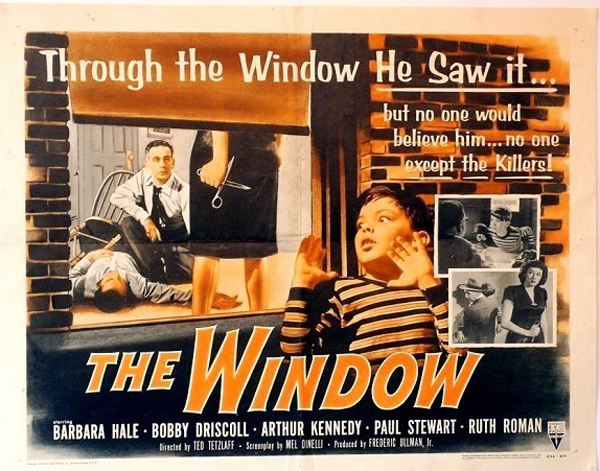This image is an advertisement for an old movie titled "The Window," likely from the 1950s or 60s, reminiscent of a fifties noir or B-movie style. The poster is predominantly in black, orange, and white, lending it a striking, dramatic tone. Centered in the image is a chilling scene viewed through a partially-drawn roller shade of a window. A young boy wearing a striped shirt stands horrified outside the window, witnessing a crime. Inside, a dead man lies on the floor, seemingly fallen from an overturned chair, and another man kneels over him, looking up anxiously. The focal point is a woman's lower body, only visible from the waist down; she wears a black skirt and holds a pair of scissors behind her back, presumably the murder weapon. 

The tagline on the poster reads, "Through the window he saw it, but no one would believe him. No one except the killers." There are also two small inset black-and-white stills from the movie, one showing the boy in conversation and the other depicting the woman with the scissors. The bottom of the poster lists the cast: Barbara Hale, Bobby Driscoll, Arthur Kennedy, Paul Stewart, and Ruth Roman. It also includes credits for the director, Ted, the screenplay by Mel O'Donnell, and is produced by Frederick somebody Jr., though these names are somewhat difficult to read.